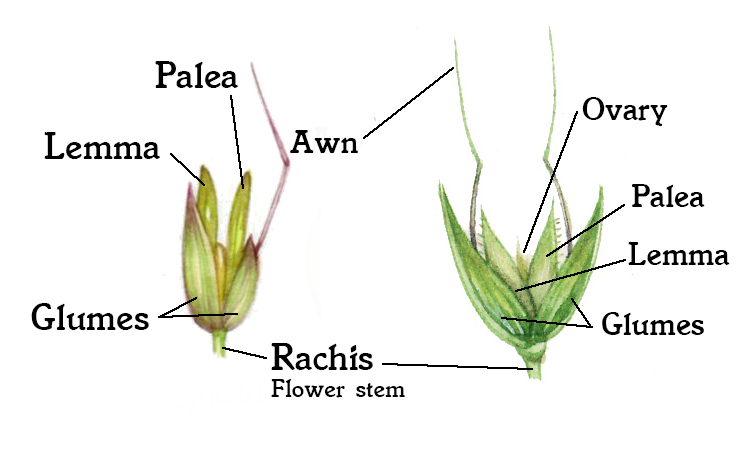In this intricate botanical illustration, labeled parts of two plants are depicted with remarkable detail. On the left side, the drawing primarily features green and yellow hues showcasing various leaves. Within this section, key terms are annotated in black text. Notably, the word "GLUM" is positioned toward the bottom, while "LEMA" (spelled L-E-M-M-A) is situated at the top. Another term, "PALEA" (spelled P-A-L-E-A), is also included. Prominently, a purple element extends from the top of this section, adding a striking contrast.

In the center of the image, the term "RACHIS" (spelled R-A-C-H-I-S) appears next to "flower stem," directing the viewer’s attention to the stem of the plant on the left. Moving to the right side of the illustration, the word "AWN" (spelled A-W-N) is clearly marked at the very top, indicating a part of a stem that showcases a blend of purple and green colors.

The right-hand plant is primarily green with white-tipped edges. Various other parts of this plant are labeled in black text for clarity. "OVARY" directs to the central part of the plant, while "PLAA" also points toward the middle. Additionally, another "LEMA" annotation identifies one of the leaves. The term "GLUMS" (spelled G-L-U-M-S) indications parts of both left and right leaves.

Overall, this detailed illustration serves as an informative guide, highlighting and naming the various anatomical structures of these botanical specimens.